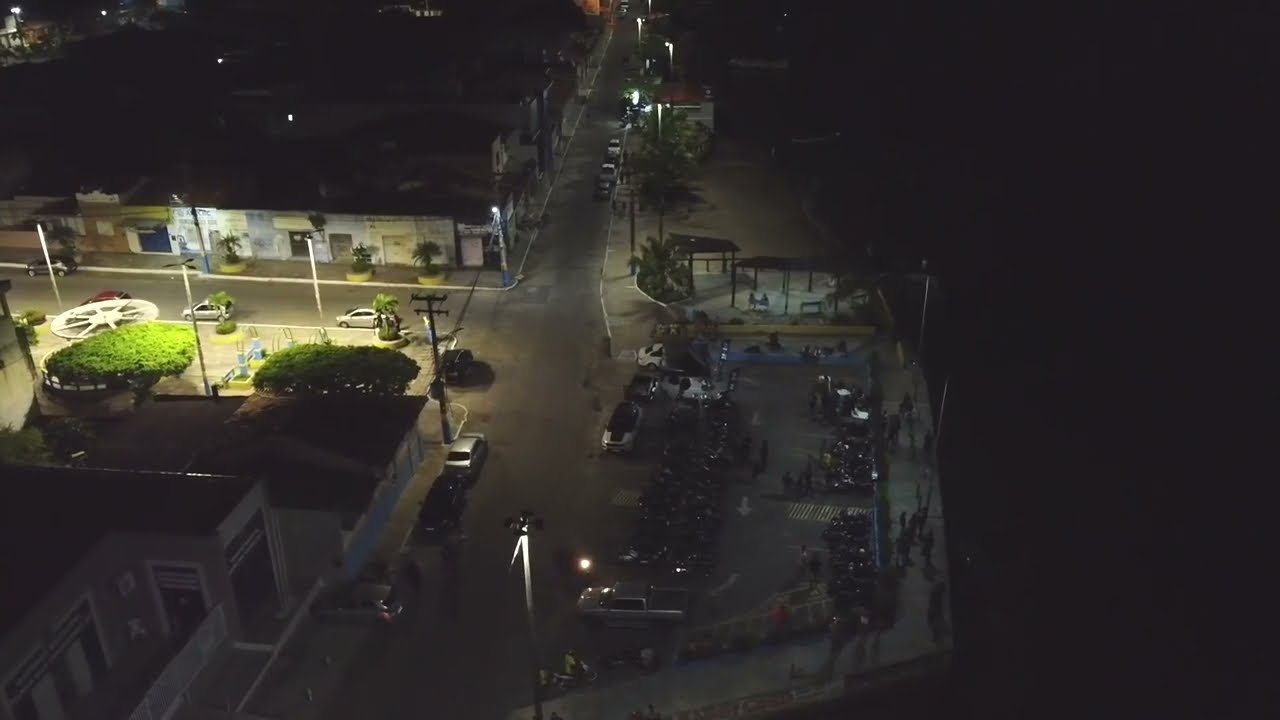This nighttime aerial photograph taken from about 15 stories high captures a dimly lit street corner illuminated by streetlights. The main street runs vertically from north to south through the center of the image. About two-thirds up, a cross street intersects and extends to the left. The far side of this cross street features a single-story building, likely a row of shops, partially revealed by streetlights. Visible are doorways and possibly signs, though details are unclear. Well-trimmed bushes line the near side of the cross street, suggesting a maintained area. To the right of the vertical main street lies a parking area, likely for dimly visible businesses.

The right third of the image dissolves into complete darkness, possibly indicative of water, as suggested by the lack of visible structures and the presence of a concrete pathway with pedestrians adjacent to this black expanse. This pathway features barriers and hints at nighttime outdoor activity. Adjacent to this area is a large, sparsely lit parking lot with directional arrows showing drive-through pathways. The photograph, taken from a three-quarter angle, also displays parked cars and potted plants along the sidewalks, reinforcing the impression of a storefront district. The overall scene combines urban elements with contrasting light and dark areas, creating a scene of quiet nocturnal ambience.